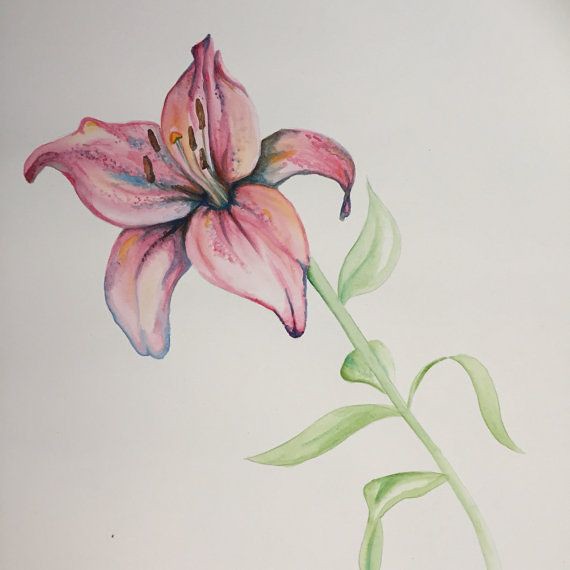This is a detailed and vibrant drawing or watercolor painting of a flower, most likely a lily. The flower is depicted with five pink petals that exhibit a gradient of colors, transitioning from a darker pink at the base to a lighter pink towards the tips, with slight hints of orange and subtle blues and greens near the base. The petals are arranged in a swooping motion and are faintly detailed, with some petals overlapping slightly.

The stem of the flower is a light green hue and extends upwards at an angle from the bottom right corner of the image, bending towards the left. Several leaves also branch from the stem: one long green leaf twists at the bottom, flattens at the top, and curves to the left; another leaf extends to the right, curves downwards, and points slightly to the right; and a few small leaves emerge further up the stem, ending with one on the right that angles upward and outward.

Crowning the stem is the flower itself, prominently displaying five pistils with brown tips and an additional pistil featuring an orange tip. The background is a muted gray, which contrasts nicely with the vivid colors of the flower, enhancing its delicate and graceful appearance.